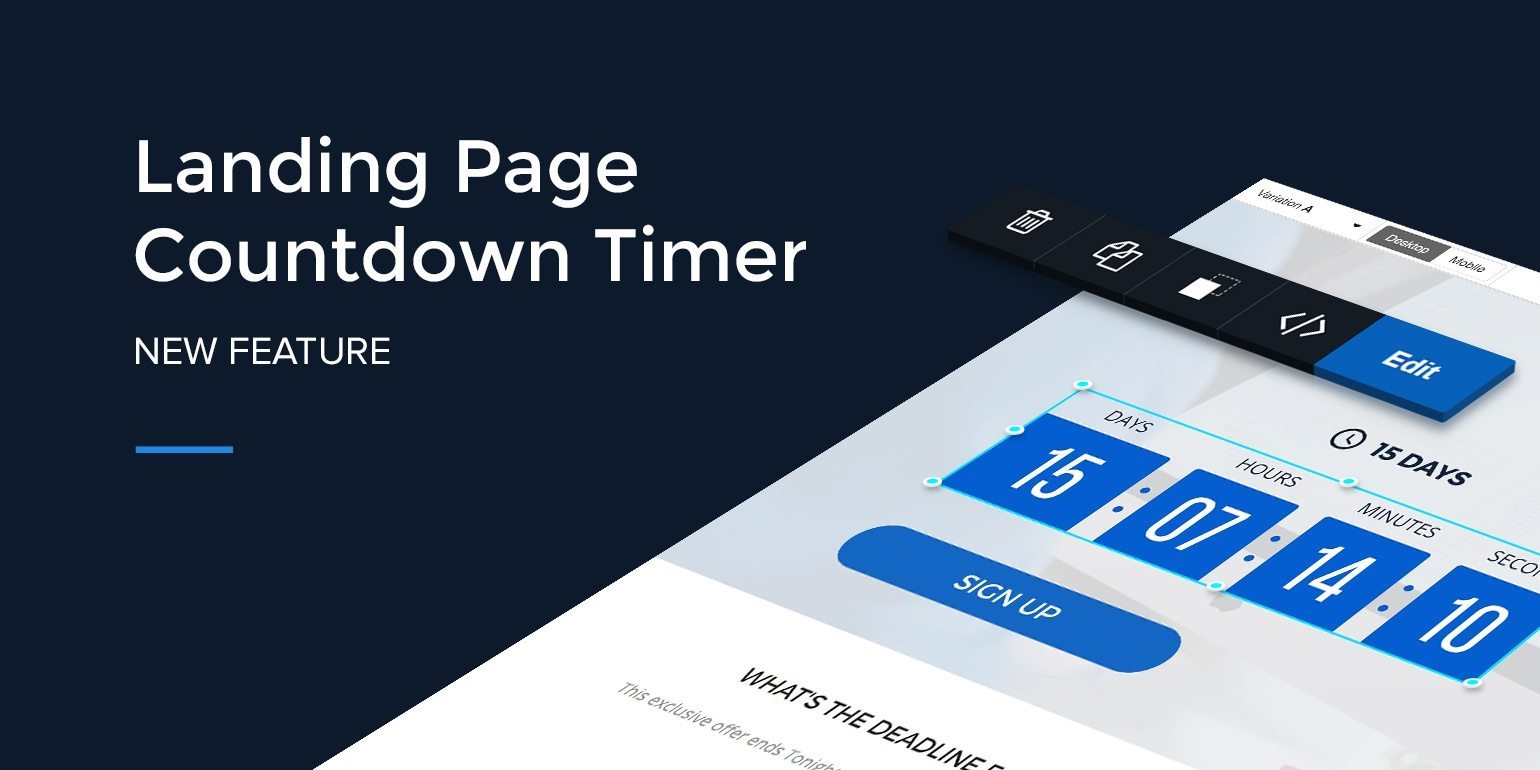The image is a product advertisement featuring a new website feature displayed on a tilted tablet or cell phone screen set against a dark blue or black background. On the right side, the text "Landing Page Countdown Timer" is prominently presented in large white letters, accompanied by smaller text "new feature" and a short blue underline beneath it.

The device screen itself showcases a user interface with utility icons, including a trash can, copy-paste, and edit buttons outlined in black and white. Dominating the screen is a countdown timer displaying "15 days" with the time units days, hours, minutes, and seconds clearly marked out below in smaller black text. Each unit has a corresponding large blue block with white numbers: "15" under days, "7" under hours, "14" under minutes, and "10" under seconds.

Below the countdown, a blue oval button labeled "Sign Up" is prominently displayed in white text. Directly beneath this button is a white text box with the phrase "What's the deadline" partially visible, and the rest of the writing is cut off. An additional, partially legible sentence follows, suggesting an exclusive offer ending soon, though the exact details remain blurry and unreadable.

The overall composition guides the viewer’s attention from the countdown timer and sign-up button to the new feature announcement, creating a visually engaging and informative depiction of the product's capabilities.